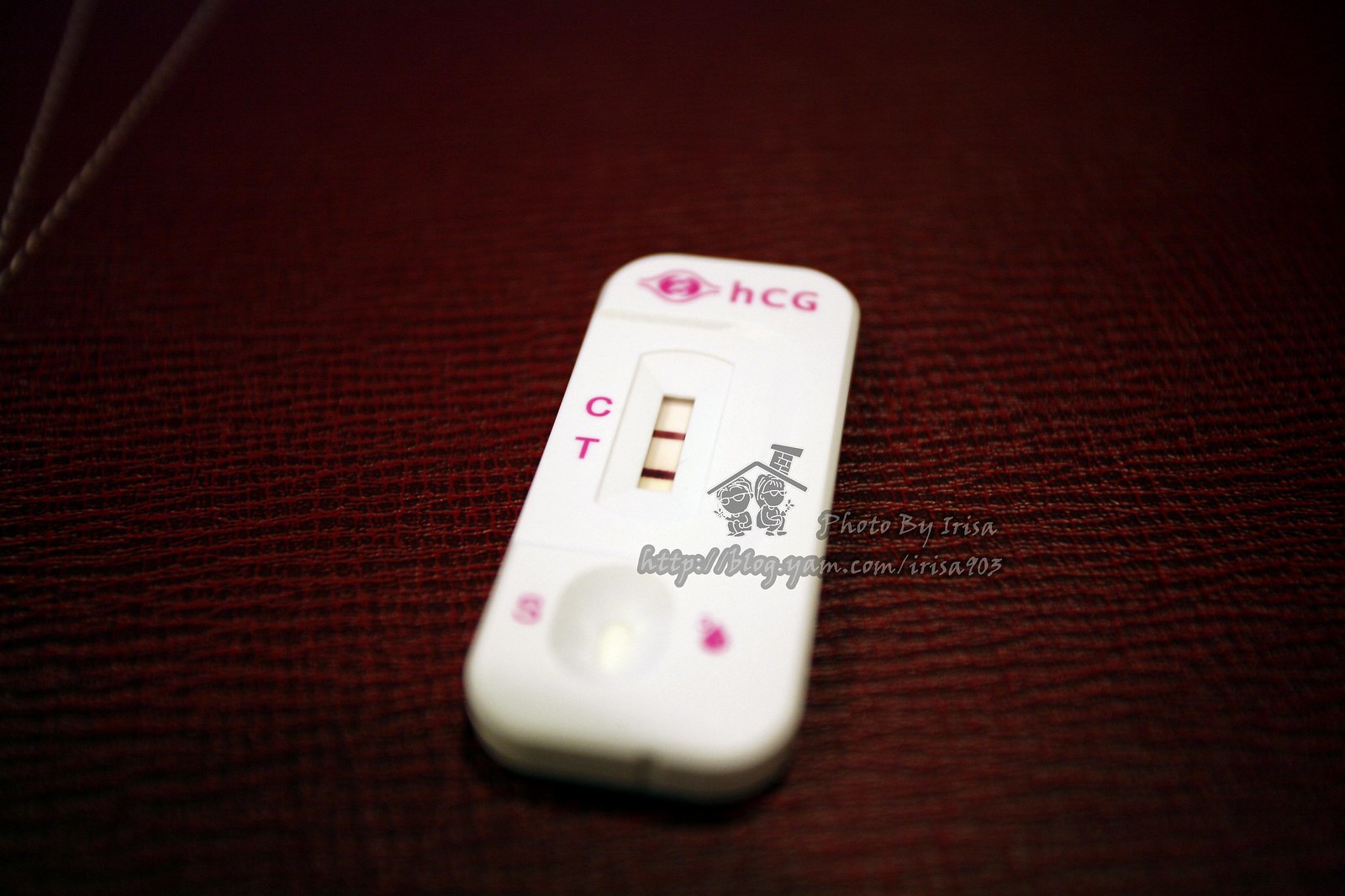A detailed photograph of a COVID-19 rapid test, which is watermarked with "Photo by Irisa" and the text "blog.yam.com, Irisa 903". The test, branded HCG, clearly indicates a positive result with two distinct lines at markers 'C' and 'T'. According to the testing guidelines, a single line at 'C' would denote a negative result, but the presence of lines at both 'C' and 'T' confirms infection. The test also features an 'S' at the lower part, which marks the spot where the sample is applied. The photograph was taken on a red carpet, adding a notable background to the image.